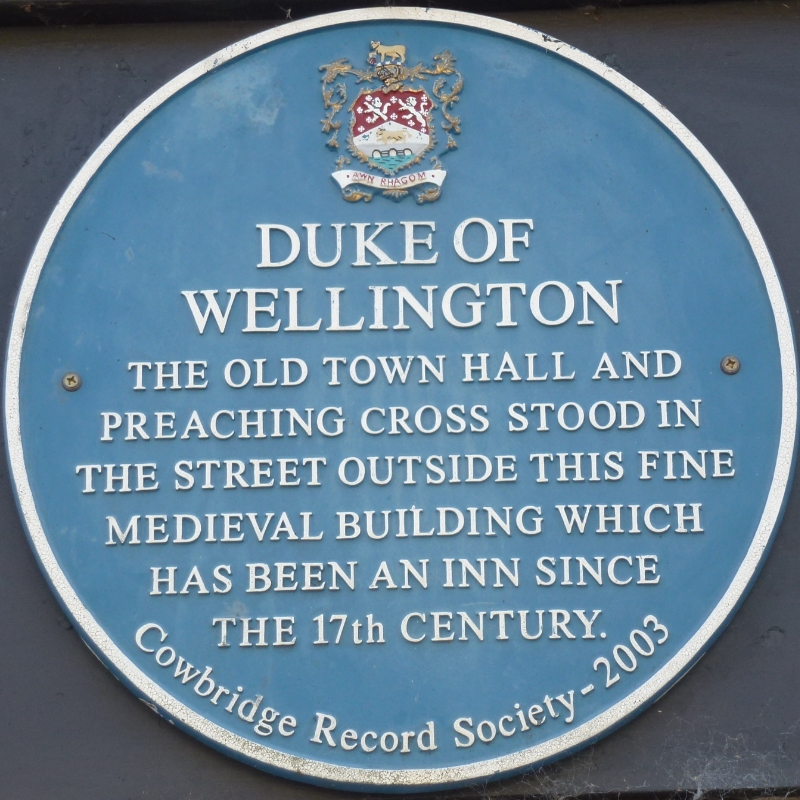The image depicts a horizontally rectangular historical marker set against a blue background, featuring an oval plaque affixed with two Phillips screws on the left and one on the right. The plaque appears to be made of metal and includes a multicolored family coat of arms at its top, which has red elements and possibly two lions, though specific details are indistinguishable. The coat of arms might include tigers on either side. Below the crest is white text that recounts significant historical information: "Duke of Wellington. The old town hall and preaching cross stood in the street outside this fine medieval building which has been an inn since the 17th century." At the very bottom of the plaque, the text reads, "Cowbridge Record Society, 2003," indicating the organization responsible for the marker.